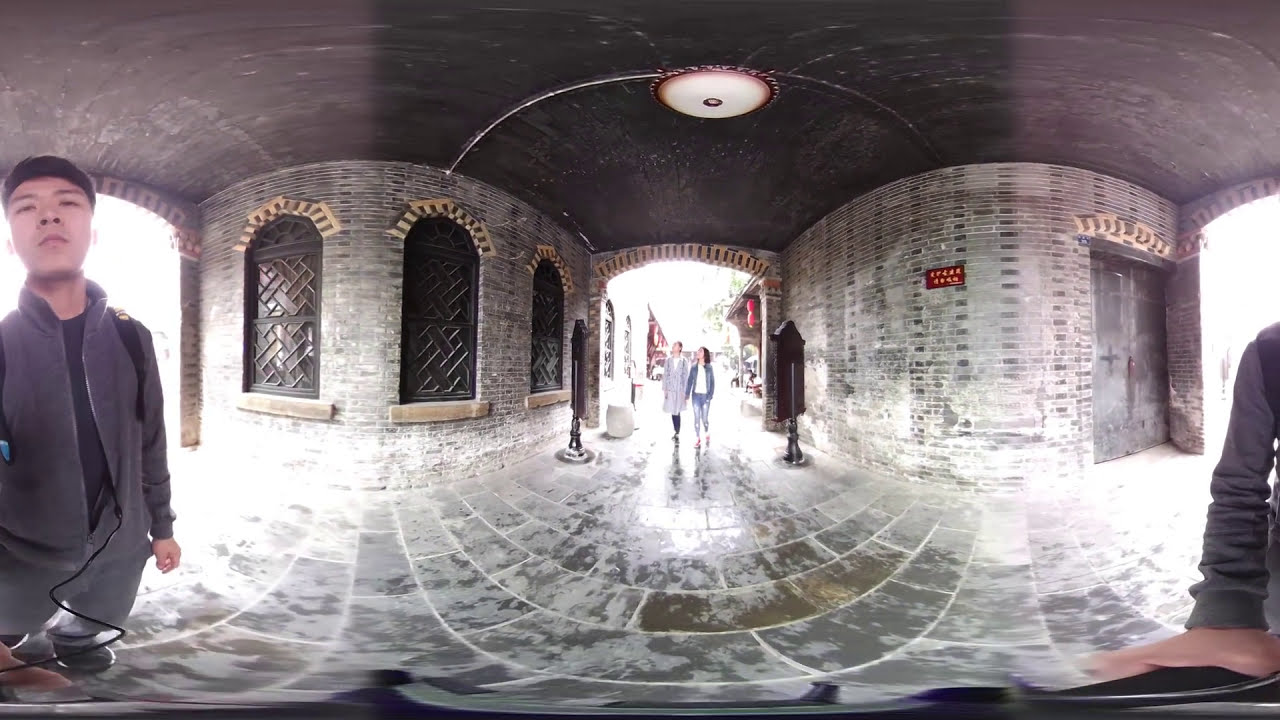The image portrays the interior of a covered tunnel or passageway, likely a popular tourist location. The setting features grey tiles and bricks, with a black ceiling adorned by a single round dome light. The ground consists of large rectangular stone pavers with white grouting, giving off a slightly medieval ambiance. In the central background, an open archway is flanked by two areas with distinctive features: three arched, beveled windows with stone ledges on the left, and a closed door on the right.

The central figure in the photograph is an Asian man in his early 30s, captured via a selfie on the left side of the frame. He wears a long-sleeved gray jacket over a black shirt and greyish shorts, with a shoulder strap visible on his left shoulder. His attire includes what appears to be a blue vest and blue pants along with a backpack. The man, with short brown hair, slightly tilts his head back, revealing a view up his nostrils. His right arm extends to the far right side of the image, holding the camera. 

This image features an edited 360-degree effect, creating a fishbowl appearance that connects the left and right sides of the photo seamlessly. Natural light filters into the enclosure, hinting at daytime, although the exact source of the light remains outside the photo. In the dim background, several other tourists traverse the passageway, suggesting the bustling nature of the location. A partially visible sign with text and a rough cave-like darkness further contribute to the intriguing yet mysterious atmosphere of the setting.